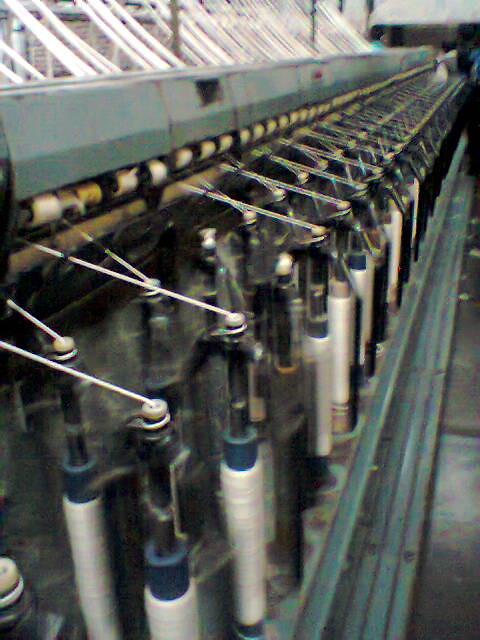The photo appears to be taken indoors, showcasing a complex piece of machinery, potentially part of an electronic assembly line or the inner workings of a device such as a keyboard. Dominating the image are rows upon rows of repetitive structures: white cylindrical rods with blue tips, from which dark rods with white tips protrude. Interspersed among them are darker rods with varying white or blue tips, all meticulously aligned in multiple rows both in the foreground and background.

Thin white strings or wires emanate from the tips of these rods, connecting to another section of the machinery, which shows what seems to be a series of keys or switches. These rods and keys are linked by numerous strings, emphasizing the intricacy of the setup. Beyond this assembly, a mysterious gray metal piece overlays the keys, and more white strings can be seen extending towards a further part of the mechanism, reaffirming the complexity and precise design of the machinery.